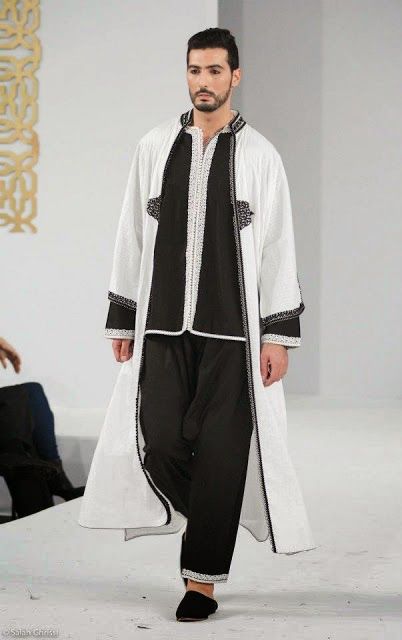The image depicts a man, possibly of Middle Eastern descent, confidently modeling a fashion ensemble down a white runway at a fashion show. He has short black hair and short black facial hair, including a mustache and beard, and maintains a neutral to serious expression. He is adorned in a long, white robe with black trim that drapes almost to his feet, revealing black pajamas underneath. The black pants feature white trim at the hemline, and the black top has white trim accents. His hands rest by his sides as he walks in black slippers. The background is composed of pure white walls, with a vertical strip of gold symbols visible in the upper left corner. Additionally, the left side of the image shows a person's crossed legs clad in black slacks, suggesting an audience member intently watching the runway.